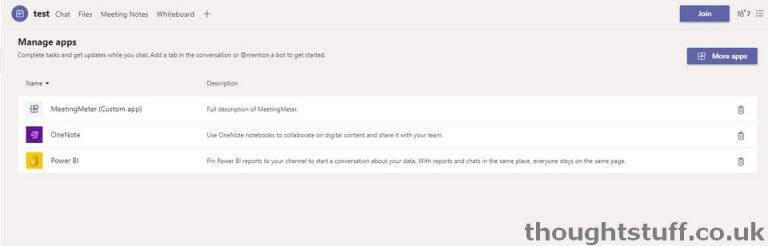The image displays a test website with a predominantly gray background. In the upper left-hand corner, the word "Test" is prominently displayed in dark black text beside a blue circular icon with a square in the center. Adjacent to "Test," there are tabs labeled "Chat," "Files," "Meeting Notes," and "Whiteboard," followed by a plus sign.

To the right, there is a purple "Join" button, accompanying a small, barely legible image that possibly displays the number 46 or 16. Directly below "Test," the phrase "Manage Apps" is written in a dark color, followed by text urging users to "Complete tasks and get supplies while you chat."

Further down, there's an instruction to "Add a tab in the conversation," although the subsequent text is hard to read. However, it does mention "to get started." Below this, there is a category labeled "Name" with a drop-down menu. Next to it, there is a section titled "Description," and a "More Apps" button located on the right side within a purple bar featuring a white square icon.

Below the "Name" category, a list follows with items such as "Meeting Master," along with mentions of "Note" and "Power." Each item is accompanied by an image to the left and a brief description underneath. To the right of these descriptions, there appears to be an icon resembling a trash box.